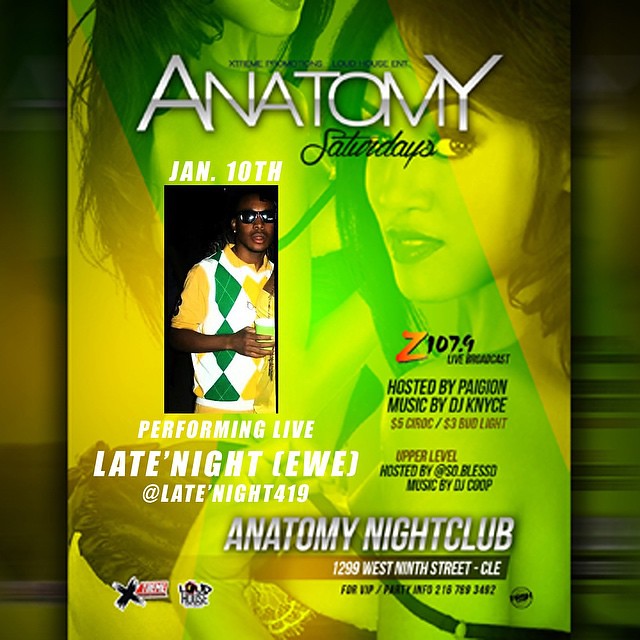The advertisement banner for Anatomy Nightclub features a sultry, green-tinted background showcasing two scantily clad women. On the right side, a mid-twenties Caucasian woman looks back over her left shoulder, wearing a low-cut top with the strap falling off her shoulder. To the left, another woman with dark hair and dark eyes stands with her hair flowing, similarly dressed in a low-cut top as she adjusts the strap. The entire background has an eerie green and yellow filter overlay.

Prominent at the top of the banner, large grey and white text announces "Anatomy," with the word "Saturdays" in black underneath. On January 10th, there will be a live performance by Late Night Lou or EWU, mentioned twice as performing at "Late Night 419." Below this, a photograph of an African-American man wearing sunglasses, a yellow sweater with a green pattern, and yellow pants is displayed. It highlights that the night features a live broadcast by Z107.9, hosted by Padjohn with music by DJ Nice. Beer prices are listed as $5 for Ciroc and $3 for Bud Light.

Further details include the Anatomy Nightclub logo at the bottom along with the address: 1299 West 9th Street, Cleveland. There are a couple of small logos, likely reading "Loud House" and "Extreme." The bottom of the advertisement provides contact information for VIP and parties, stated as very small and hard to read.

Overall, the leaflet or poster vividly combines a sensual and dynamic vibe, promoting an exciting Saturday night event at the Anatomy Nightclub.